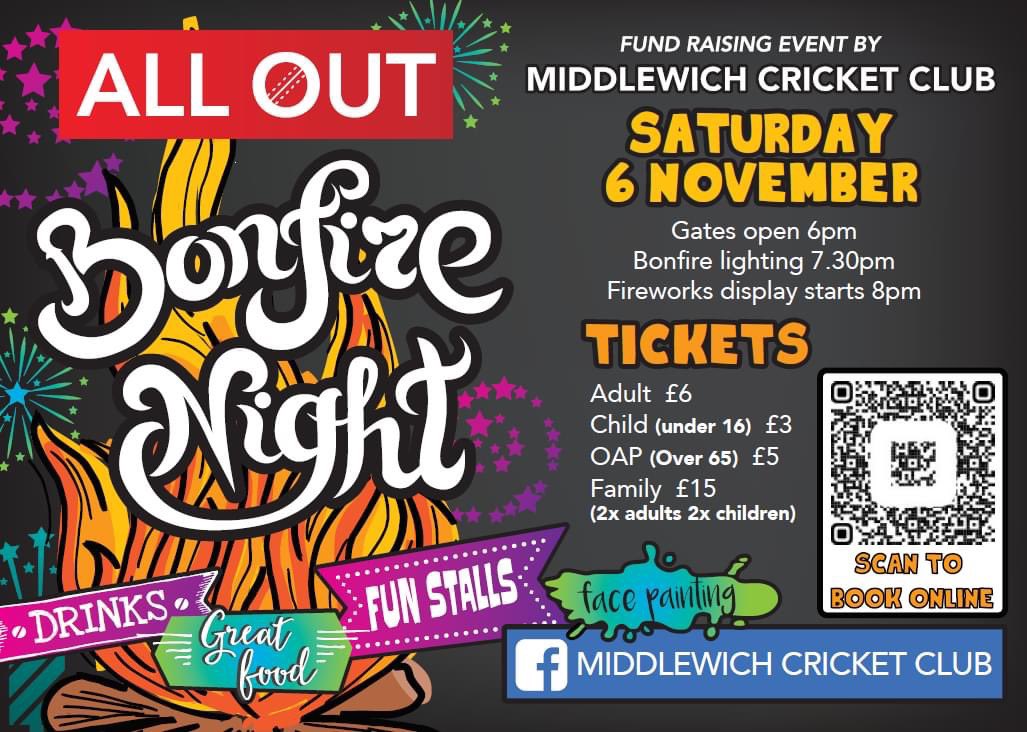This is a detailed and vibrant Facebook advertisement for the Middlewich Cricket Club’s upcoming event, "All Out Bonfire Night." The background is predominantly black, accentuated by an array of colorful fireworks in green, purple, and star shapes, creating a festive atmosphere. Prominently displayed at the top right is a red rectangle with bold white text declaring, "All Out." Just below, in a stylish, almost handwritten font, "Bonfire Night" is set against a graphical bonfire with vivid red, orange, and yellow flames shooting skyward.

Beneath the bonfire graphic, two colorful boxes provide further details: a purple box with white text offering "Drinks", "Fun Stalls", and a green box with cursive white text promoting "Great Food." To the left, more crucial details unfold in clean white and yellow text. The event is tagged as a "Fundraising Event by Middlewich Cricket Club," scheduled for Saturday, 6th November. Timings are clearly listed: gates open at 6 p.m., the bonfire lighting is at 7:30 p.m., and the fireworks display starts at 8 p.m.

Ticket prices are transparently shared: Adults £6, Children under 16 £3, OAPs over 65 £5, and Family tickets (for two adults and two children) are £15. Highlighted in a green and blue paint splat are additional attractions like "Face Painting." There’s also a QR code on the left under the "Scan to Book Online" instruction. The bottom of the advertisement proudly announces the Middlewich Cricket Club as the event organizer with a Facebook logo directing visitors to their social media page for more information.